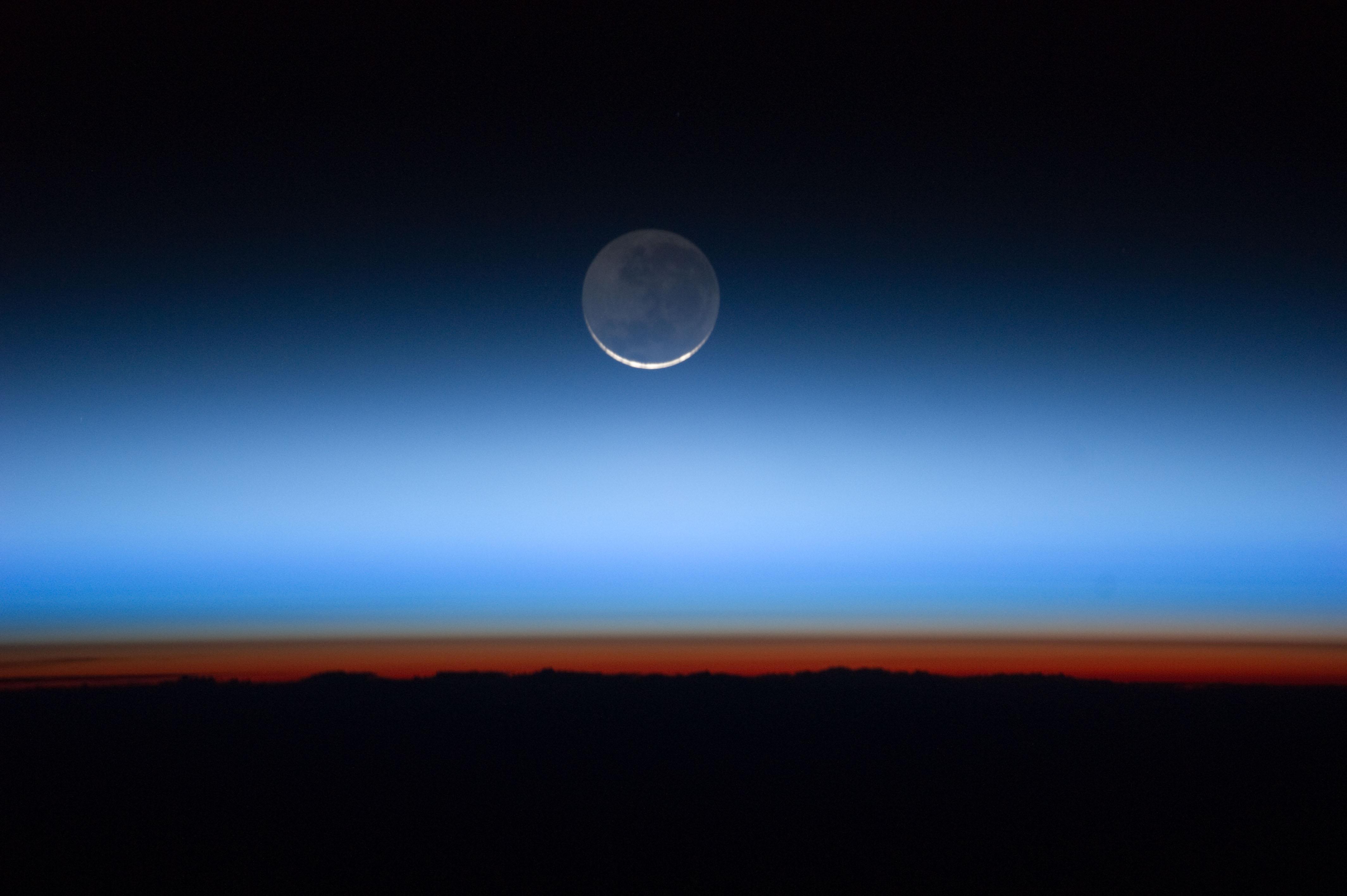This detailed color illustration captures a striking desert moonscape at dusk. Set in a landscape orientation, the image showcases a vast, barren desert that stretches across the foreground in dark silhouette from the bottom left to the bottom right. Above this silhouette, a narrow horizon glows in brick red, topped by a lighter gold band. Ascending from the horizon, a gradient of light blue fades to darker shades, reaching up to meet the pitch-black night sky that crowns the scene. Dominating the center upper portion of the image is a large, shadowed moon with a bright white crescent glowing along the top edge. The scene exudes a serene yet desolate beauty, with the clear, starless sky enhancing the sense of infinite space.